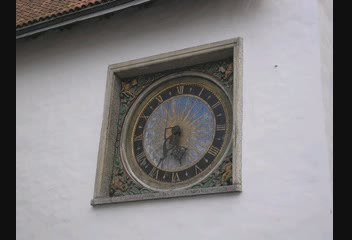This photograph showcases a wall clock that appears to be seamlessly embedded within a square indentation in the wall. The clock itself features a circular frame with an elegant analog face. Roman numerals mark each hour, and the clock hands are intricately designed with ornate details. At the center of the clock, there is a distinctive sun motif. Surrounding the circular timepiece are exquisite floral patterns that extend to fill the square space, blending artistry and functionality into a harmonious design.